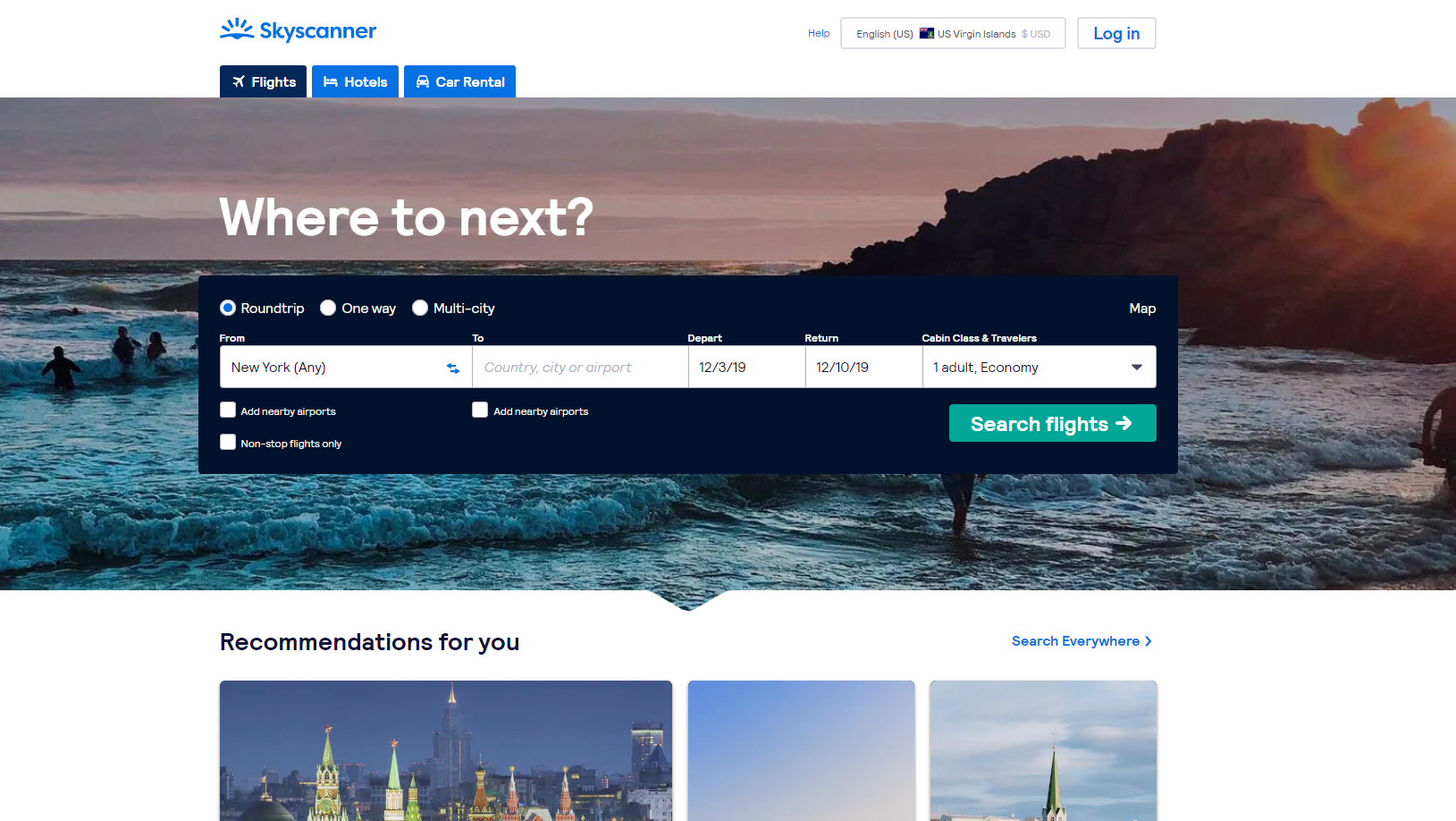The image showcases the user interface of the Sky Scanner website, featuring a prominently displayed white top border that includes a blue logo of the sun rising over the horizon, accompanied by the text "Sky Scanner". Directly below, there is a language selection bar displaying options such as "English (U.S.)", and preferences for the "U.S. Virgin Islands" and "U.S. Dollar (USD)". Nearby, a white 'Login' button is visible.

Further down, the navigation menu presents options for "Flights", "Hotels", and "Car Rentals". The background of the webpage is illustrated with a serene beach scene, characterized by a purple sky and a distant, towering hill densely covered in forest.

Overlaying this scenic backdrop is a search interface featuring options such as "Round Trip", "One Way", and "Multi-City". The search fields prompt users to enter details like departure from "New York, any", destination to "Country, City, or Airport", with specified travel dates of departure on "12-3-19" and return on "12-10-19". Additionally, it specifies travel class and passengers as "One Adult, Economy". A prominent rectangular button labeled "Search Flights" invites users to initiate their search.

Below this section, the webpage offers personalized recommendations with three thumbnail images highlighting various travel options.